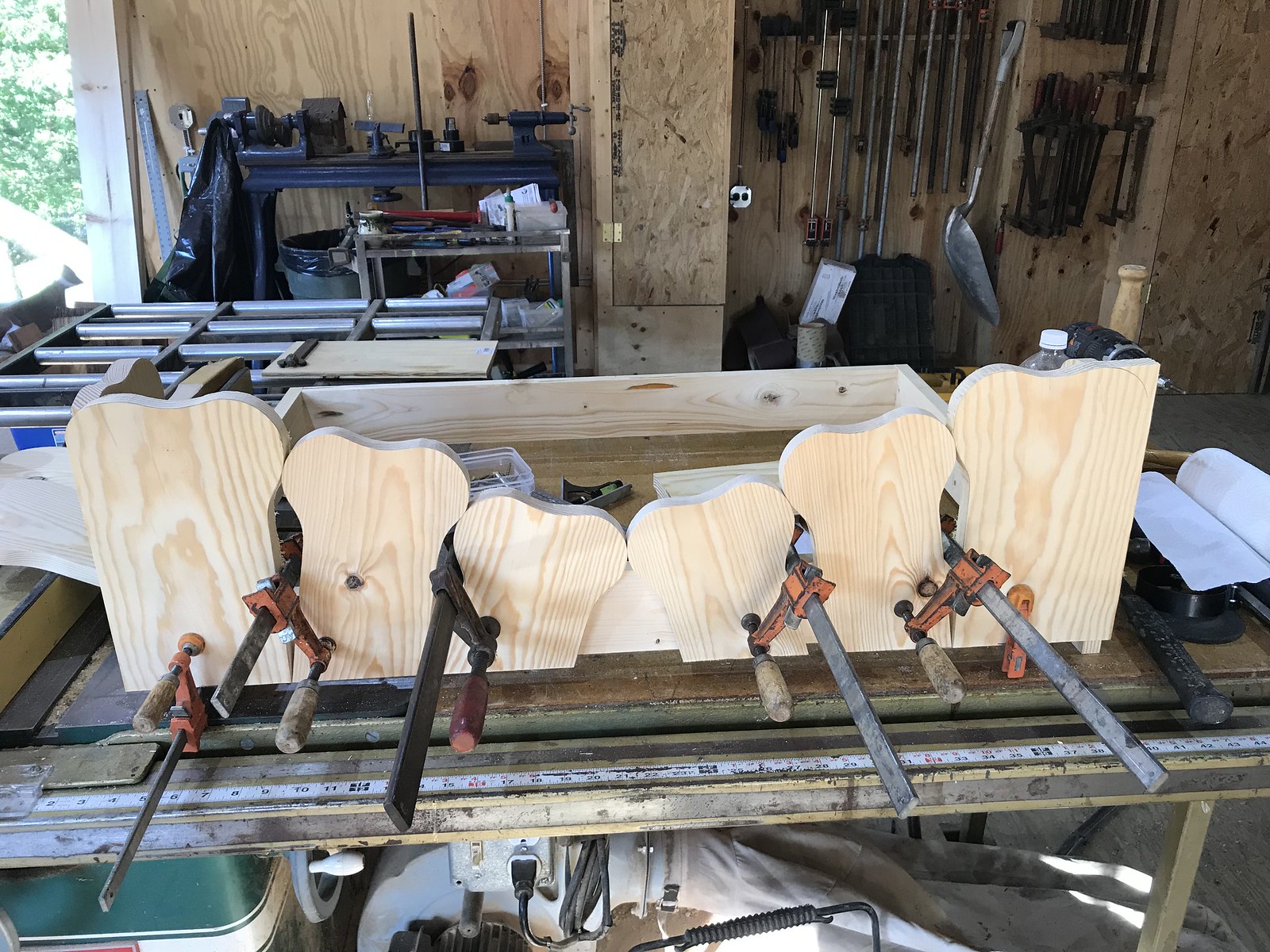In this detailed color photograph of a converted garage workshop, the background features a light-colored wooden wall adorned with an array of hanging tools, including a prominent metal snow shovel. Central to the image is a substantial metal workbench topped with wood, its front edge marked with a long measuring ruler or tape measure integrated into the table's surface. Securely held in the vise on the bench are six pieces of light brown wood, carefully shaped at their ends to resemble dog biscuits or bones. The sophisticated arrangement for woodworking includes a handsaw with a metal gripper and a line extending from the top. Surrounding the workspace, a variety of hand and lawn tools are meticulously organized on a metallic storage unit, and an open doorway in the upper left corner reveals lush green trees outside, further complementing the workshop's industrious ambiance. Below the worktable, a power outlet is visible, equipped with a black plug connected to an extension cord, emphasizing the electrical needs of the workshop. The scene is devoid of any people, focusing entirely on the detailed setup and craftsmanship in progress.